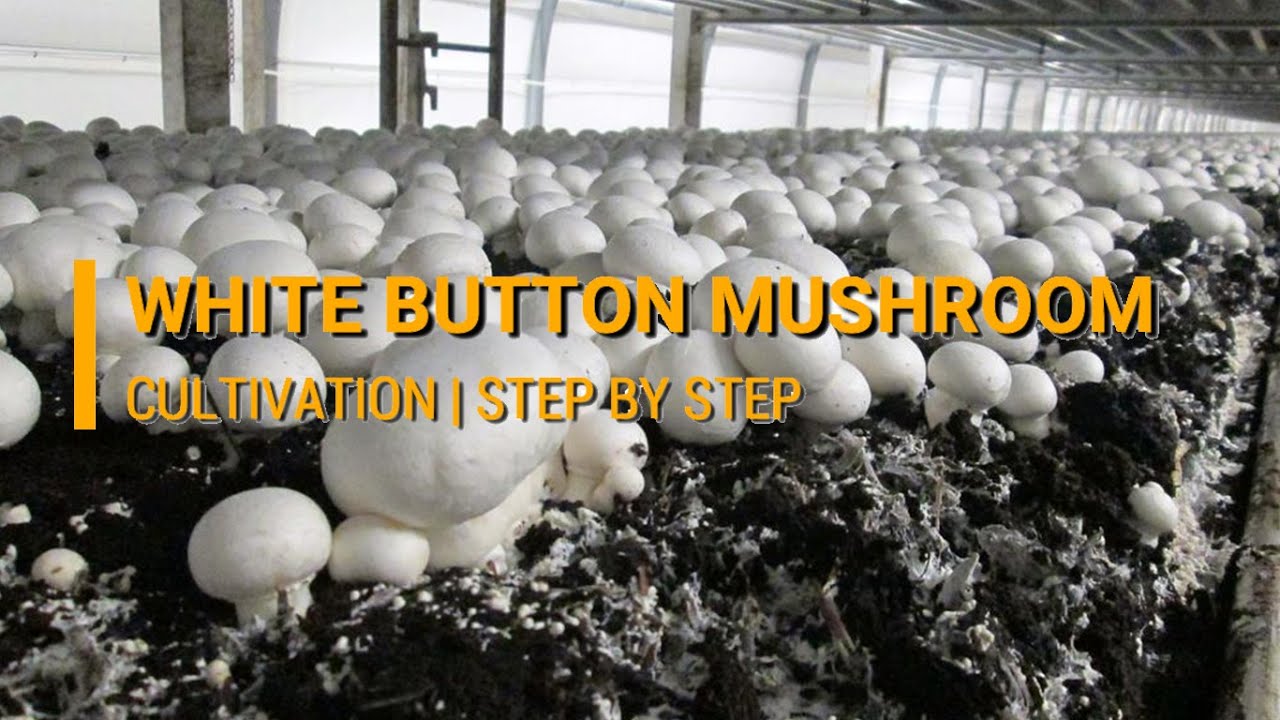The black and white image showcases a vast indoor farm or greenhouse dedicated to growing white button mushrooms. Spreading out as far as the eye can see, the white-cap mushrooms are thriving in what appears to be rich, dark substrate dotted with mycelium. The ceiling structure and windows in the background hint at the spaciousness and industrial scale of this operation. Overlaying the entire image, vertical orange text reads "White Button Mushroom Cultivation: Step by Step," suggesting an educational or instructional purpose. The text stands out with a slight 3D effect, providing an eye-catching contrast to the monochrome background. This detailed and visually striking image serves as a comprehensive guide on mushroom cultivation.